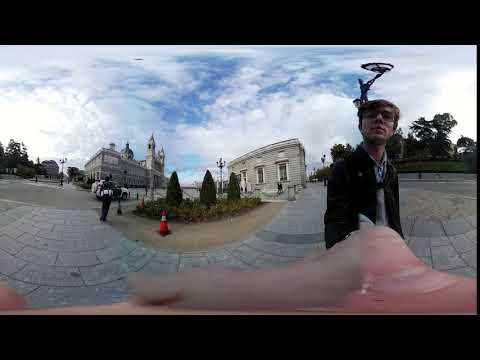This image is a 360-degree panoramic photo taken outdoors in what appears to be a city square. The photographer, whose outstretched arm is holding the camera or cell phone, is visible in the photo; they are wearing a black overcoat, a light-colored button-down shirt, glasses, and short hair. The sidewalk they stand on features a patterned, tiled granite design. 

In the center of the image, partially convex due to the panoramic effect, lies a decorative grassy patch with three small evergreen trees and a vivid orange traffic cone positioned in front of it. Just to the left, a man with a white backpack is walking towards a black and white SUV parked on the adjacent street. To the right, a man dressed in a dark blue jacket with glasses stands near a light pole, beneath which a grassy hill slopes upwards, edged by partially obscured buildings hidden by trees. 

In the background, there are two large, solid buildings made of gray or white-colored stone, suggesting durability and strength. A statue, featuring a man holding a dish in the air, is visible directly behind the man in the dark blue jacket. The sky overhead is a light blue, dotted with clouds, indicating a mostly cloudy day.